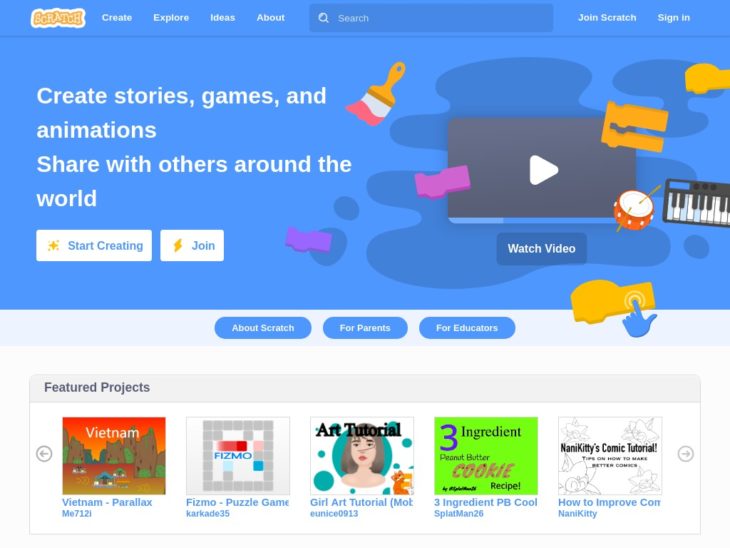This image is a detailed screenshot of the Scratch website. The logo, placed in the upper left corner, features the word "Scratch" in bold, cartoonish letters that are yellow with orange outlines. The upper part of the website has a light blue background and a navigation toolbar. This toolbar includes links labeled "Create," "Explore," "Ideas," and "About." To the right of these links, there is a search box, followed by links for "Join Scratch" and "Sign In" located at the top-right corner.

The main body of the webpage is filled with various colorful elements, including cartoonish paint brushes, puzzle pieces, a stylized drum set, and keyboards. Prominently featured in the center is a video player with a blue "Watch Video" button below it. At the top of this central section, text reads: "Create Stories, Games, and Animations, Share with Others Around the World." Below this, there are buttons labeled "Start Creating" and "Join."

Toward the bottom of the webpage, there are Featured Projects, showcasing a variety of content including "Vietnam Parallax," "Fizmo Puzzle Game," "Girl Art Tutorial," "Three Ingredient PB Cool," and "How to Improve."